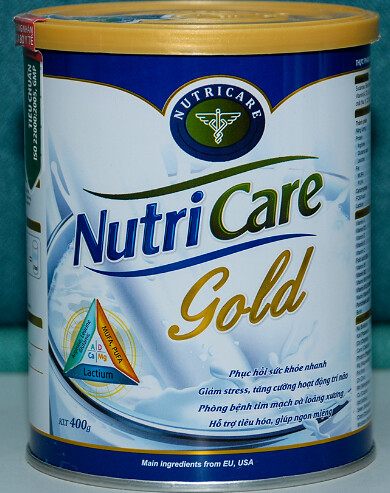The image features a close-up of a medium-sized tin can labeled NutriCare Gold, prominently displayed on a white counter, suggesting it might be in a kitchen. The can has a gold plastic lid that looks removable and a paper seal on the left side. The main body of the can is primarily white with gold edging at the top and bottom. In the center, the NutriCare logo is showcased within a blue circle and features a green oval design. The label includes various details: the main ingredients are sourced from the EU and the USA, and the packaging includes information in another language, possibly Thai. Additionally, there's a green swirling line and a triangle in one corner listing the ingredients. The can is sized at 400 grams and hints at various health benefits. The background is a light blue wall, further accentuating the clean, medical-like design of the product.